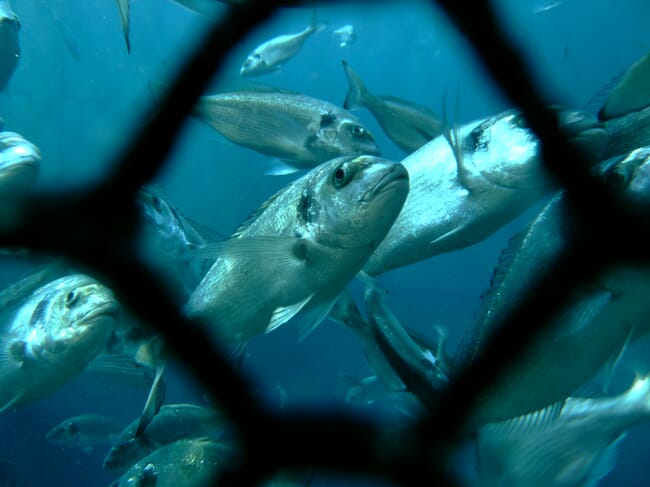The image reveals a close-up view of a fish tank or an underwater scene, with the camera lens capturing the scene through a black, hexagonal-patterned barrier, possibly resembling a cyclone fence or a grid. This obscures part of the view and extends horizontally, suggesting a continuous pattern. Several silvery fish, resembling small tuna, are visible swimming against a blue backdrop, with the light from above casting a gentle shimmer on their upper bodies. The fish, characterized by their round faces, short top fins, and paired bottom fins, are primarily moving towards the right side of the frame. The scene includes dozens of these fish, with a few prominently positioned near the lens, while the others are dispersed in the background. Additionally, there seems to be a plant or whisker-like element near one of the fish’s gills, adding a touch of the aquatic environment's detail.